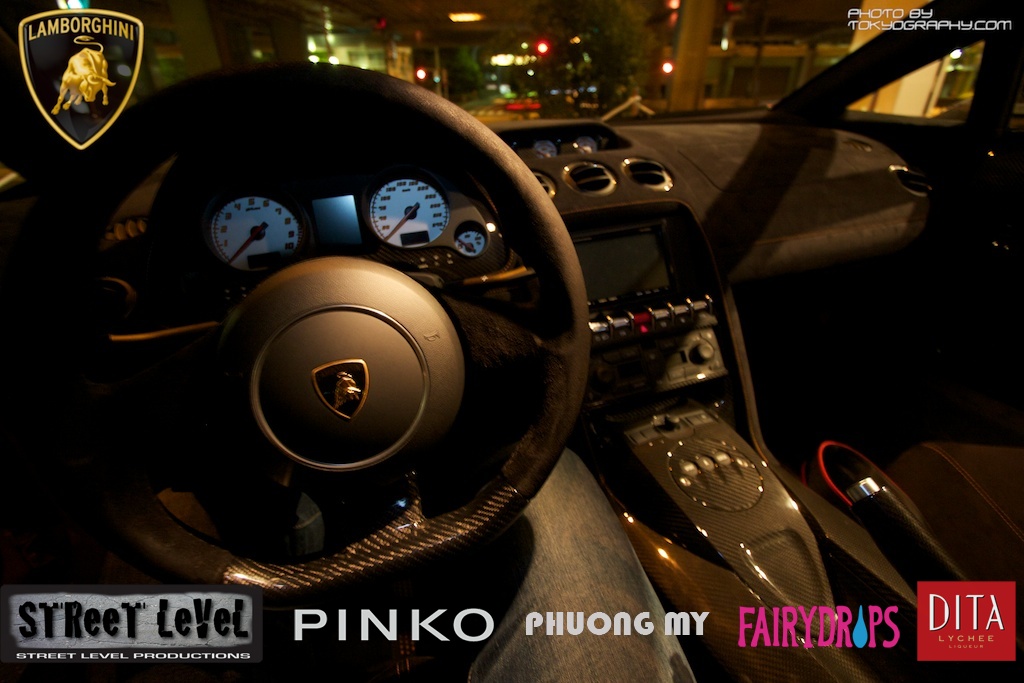This detailed photograph, taken from the driver's seat of a Lamborghini, captures the luxurious interior of the car at night. The black steering wheel prominently features the iconic Lamborghini logo at its center, and the black dashboard is accented with sleek carbon fiber trim. Visible in the lower part of the frame are the driver's legs clad in jeans, providing a personal touch to the scene. Outside the windshield, dark night skies contrast with the glow of street lights illuminating the road ahead. 

In the upper left corner of the image, the Lamborghini logo is displayed once more, emphasizing the brand's presence. The top right corner features the text "Photo by Tokyography.com" in white, giving credit to the photographer. Along the bottom, several names and logos are seen, including Street Level Productions and Dita Lychee written in white within a small red square. Though the snapshot conveys the night-time exterior setting, the detailed and well-lit interior highlights the elegance of the Lamborghini.